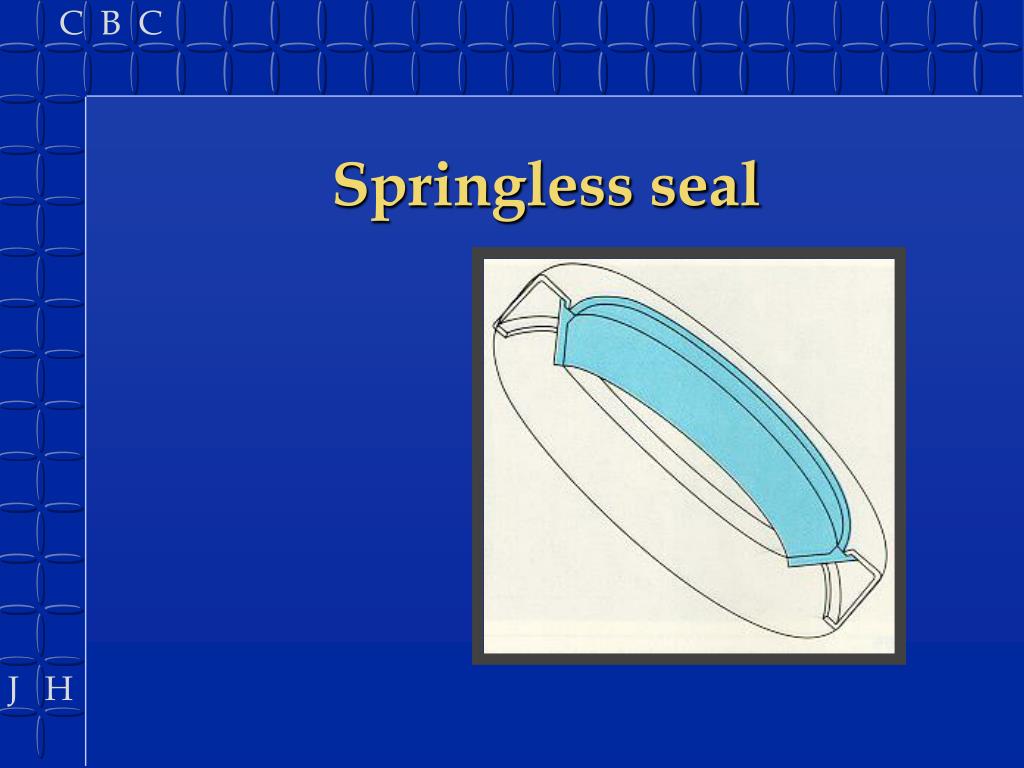The image consists of a royal blue square with a unique border along the top and left sides, featuring small squares within. In the upper left corner, the capital letters "C, B, C" are placed, while in the lower right corner, just above the border, there are white capital letters "J, H." Inside this border is another blue square. At the top of this inner square, the text "Springless Seal" is written in yellow. Beneath this text, there is a white box containing a line drawing of a product, possibly a boat or a lid’s seal, outlined in black and blue. The image appears to serve as an advertisement or diagram, with elements set at a diagonal to emphasize the details. The background and framing use varying shades of blue to create a checkered effect.